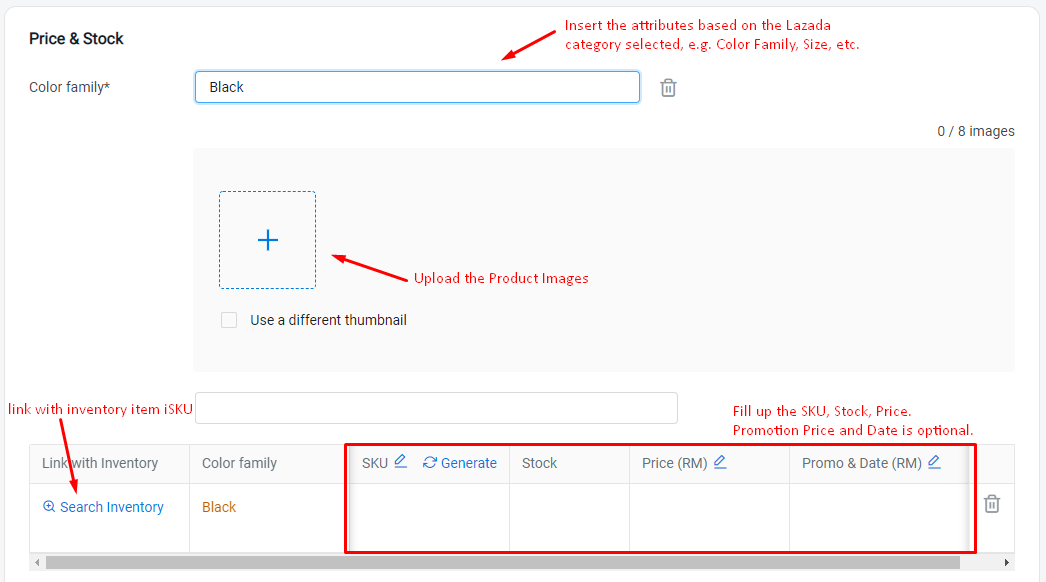The image features a detailed user interface element. Central to the composition is a white rectangular area bordered by a gray line. At the bottom, there's a horizontal scroll bar for navigation. 

In the top left corner, the text "Price and Stock" is prominently displayed. Below that, the label "Color Family" is present, adjacent to a text box with a blue border that reads "Black". A trash icon is positioned immediately to the right of this text box. Above the text box, a red arrow points towards it, accompanied by the instruction, "Insert the attributes based on the Lozada category selected, e.g. color family, size, etc."

Below this section, a light gray box is visible. Within this area, there is a blue-outlined square with a blue plus sign at its center. To the right of this, another red arrow points towards the box with the label "Upload product images". Below this, a checkbox, currently unchecked, is labeled "Use a different thumbnail".

Further down, towards the left side, there is a "Search Inventory" feature with a red arrow pointing at it, highlighting its importance.